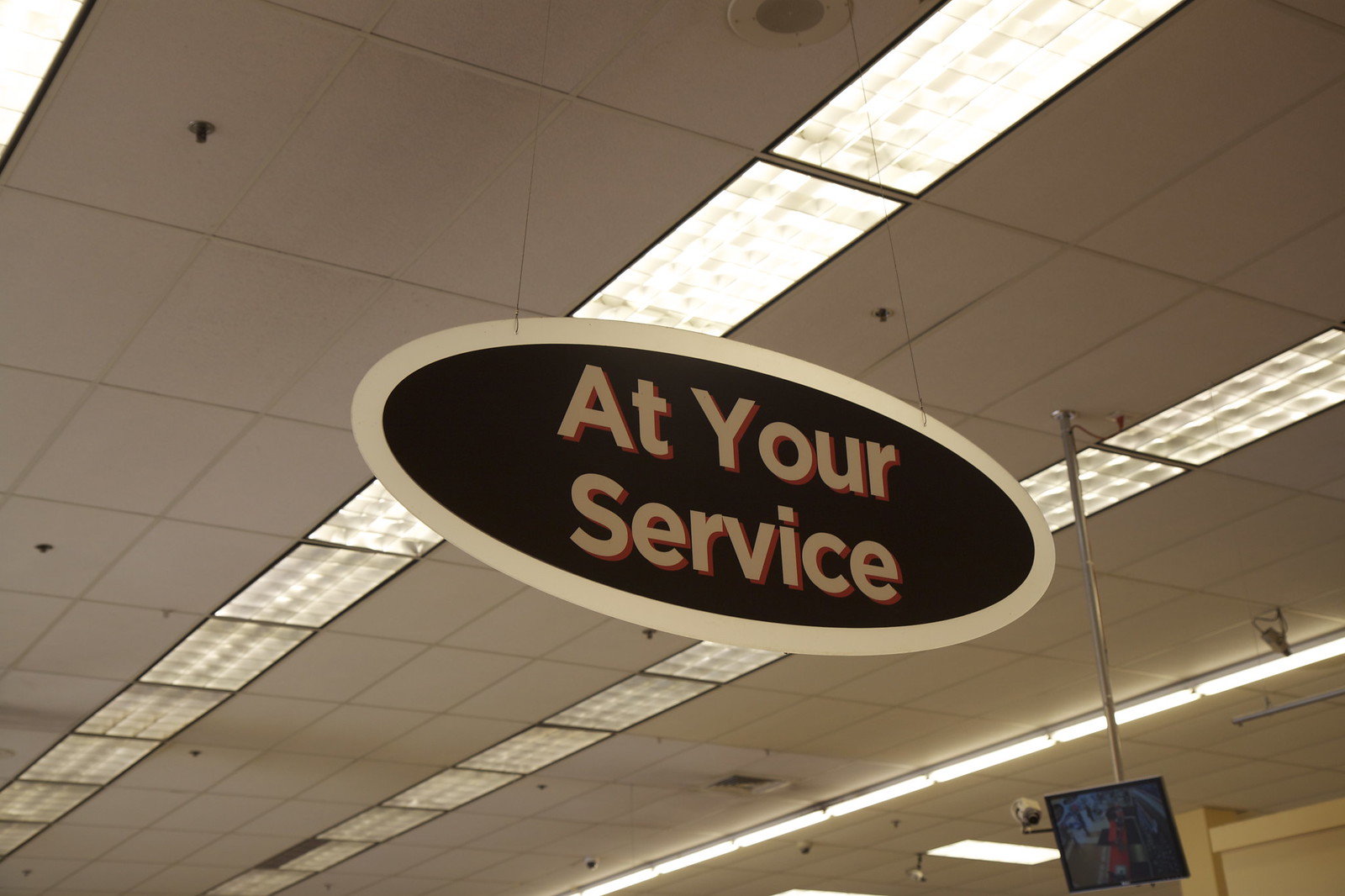This photograph, taken indoors from a low upward angle, captures the ceiling of what appears to be a department store. Dominating the scene is an oval-shaped sign, horizontally aligned, suspended from the white false ceiling by two thin strings. The sign features a beige border with a dark, possibly black interior, prominently displaying the phrase "At Your Service" in large beige or cream-colored letters. Red drop shadows add depth to the text. The ceiling is adorned with strips of fluorescent lighting running across the image, and small sprinklers dot the panels. Additionally, a stainless steel or chrome pole descends from the ceiling, terminating in a flat-screen monitor that faces left, presumably monitoring a particular area of the store. The photograph primarily focuses on the ceiling and its fixtures, with no other store details visible.